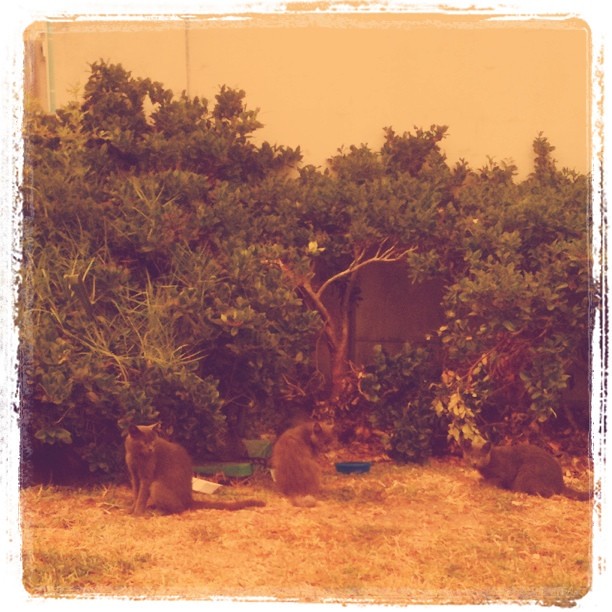In this vintage-style photograph, which appears either genuinely aged or enhanced with a sepia filter, we see a seemingly old image with torn and faded edges resembling a Polaroid from the 60s or 70s. The photo captures a backyard scene with dry, straw-brown grass and green bushes against a pale yellow wall. Three dark gray cats with slight white spotting and yellow eyes are lounging in the foreground. Two cats sit upright, one with its back to the camera while twisting to glance over its shoulder, and the other gazing off to the right. The third cat lies sideways on the grass, head cocked forward, looking directly at the camera. Scattered around are various bowls and containers, including blue and white dishes, indicating these are likely outdoor pets. The entire image exudes a nostalgic charm, emphasized by its washed-out, yellowish-peach hue and rough, streaked edges.